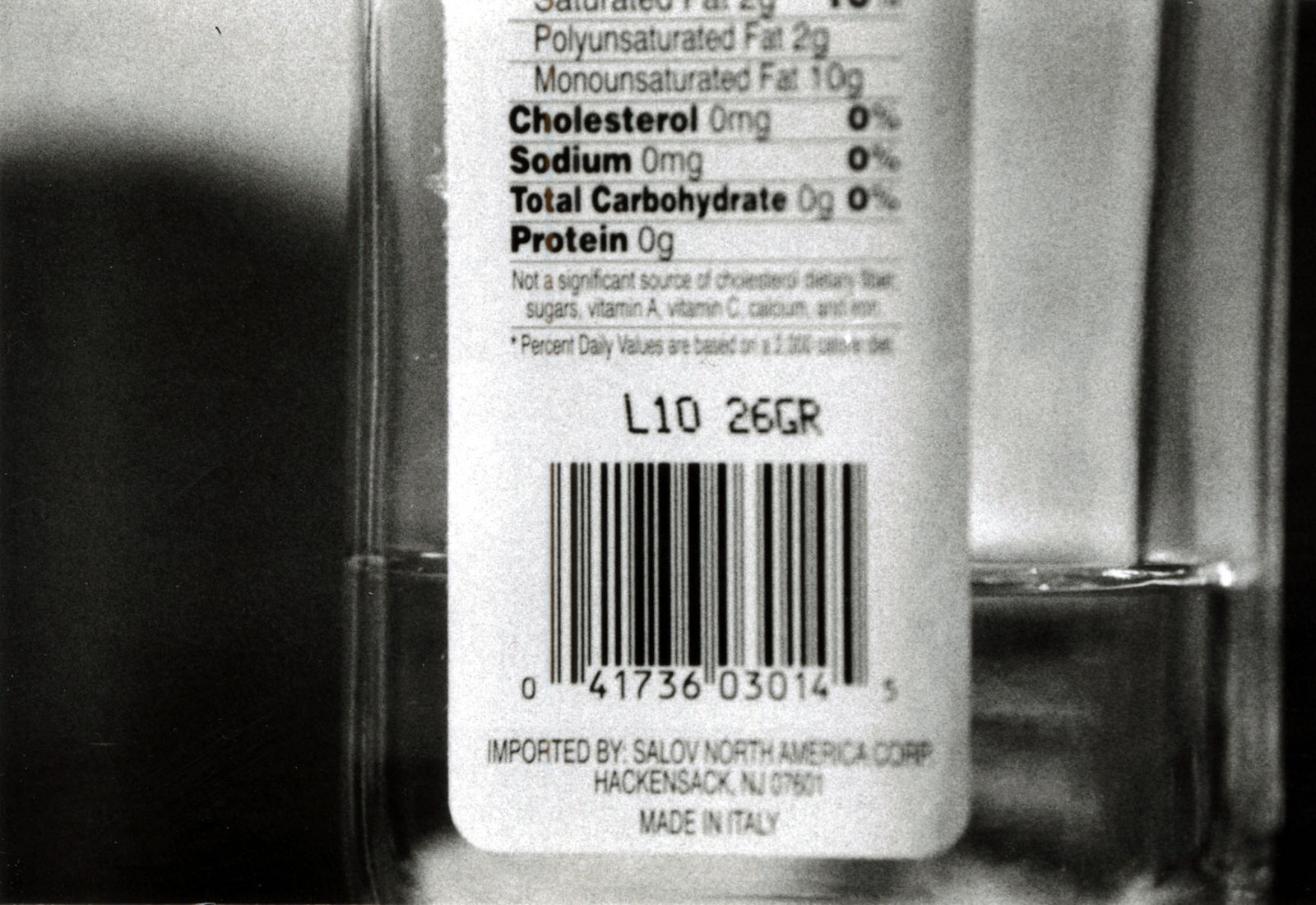This highly detailed black and white close-up image prominently features a glass bottle with a narrow shape, containing approximately a quarter of a clear liquid. The focal point is a large barcode on the bottom of the bottle’s back, with the lot number "L1026GR" positioned above it. Below the barcode, the text reads "Imported by Solove North America Corp, Hackensack, New Jersey," followed by "Made in Italy." The bottle bears a white label on its back, partially displaying the nutritional facts panel, which lists saturated fat (2 grams), polyunsaturated fat (2 grams), monounsaturated fat (10 grams), and indicates zeros for cholesterol, sodium, total carbohydrates, and protein. It also mentions that it is "not a significant source of cholesterol, dietary fiber, sugars, vitamin A, vitamin C, calcium, or iron." An asterisk notes that "percent daily values are based on a 2000 calorie diet." A white label on the front of the bottle is partially visible through the glass. The left side of the background is predominantly shadows, with a hint of light coming from the top, but it is out of focus.